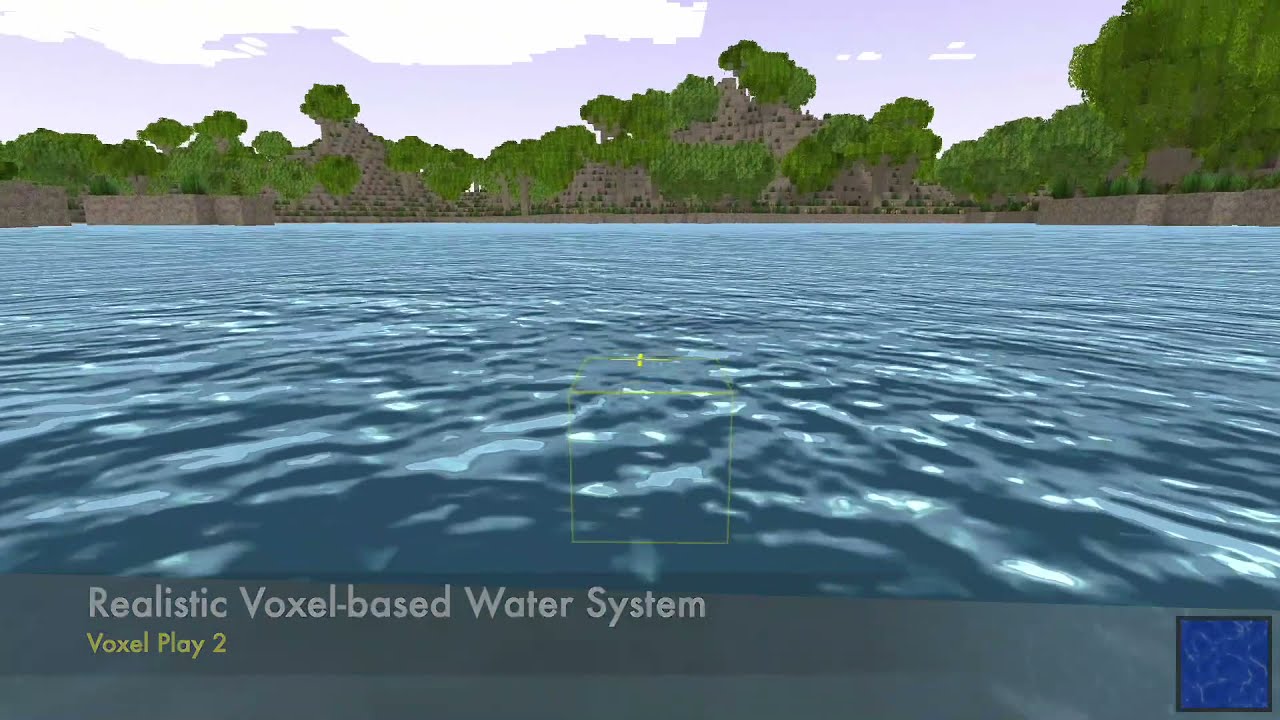The image appears to be a digital screen capture, showcasing a voxel-based visualization. Dominating the scene is a pixelated body of water, featuring dark blue, medium blue, and light blue tones designed to suggest movement. In the background, sand-colored bricks form a wall, interspersed with green trees. The ground is rendered in shades of green and brown, complementing the pixelated landscape. Above, a sky of pale purple and white hues stretches across the scene. Central to the image, a cube outlined in green or yellow lines floats prominently. Across the bottom, text reads "Realistic Voxel-Based Water System" and "Voxel Play 2" in yellow letters, emphasizing the technological focus of the visual representation. The entire scene is infused with a pixelated aesthetic, enhancing the digital, voxel-based theme.